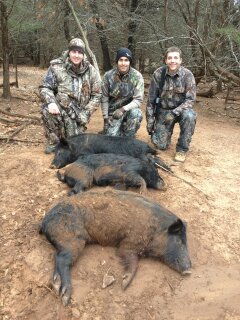In a somber woodland scene, three men dressed head-to-toe in camouflage hunting gear kneel on one knee behind their trophies: three dead wild boars. They smile at the camera, displaying their accomplishment. The wooded setting features a dirt-covered ground devoid of grass or walkways, with sparse trees and shrubs showcasing green and brown leaves in the background. The wild boars are lined up in front of the hunters, their black fur varying from pure black to black with patches of brown, possibly dirt-streaked. The ground surrounding the downed animals and hunters is entirely earthy, reinforcing the sense of desolation in the image.